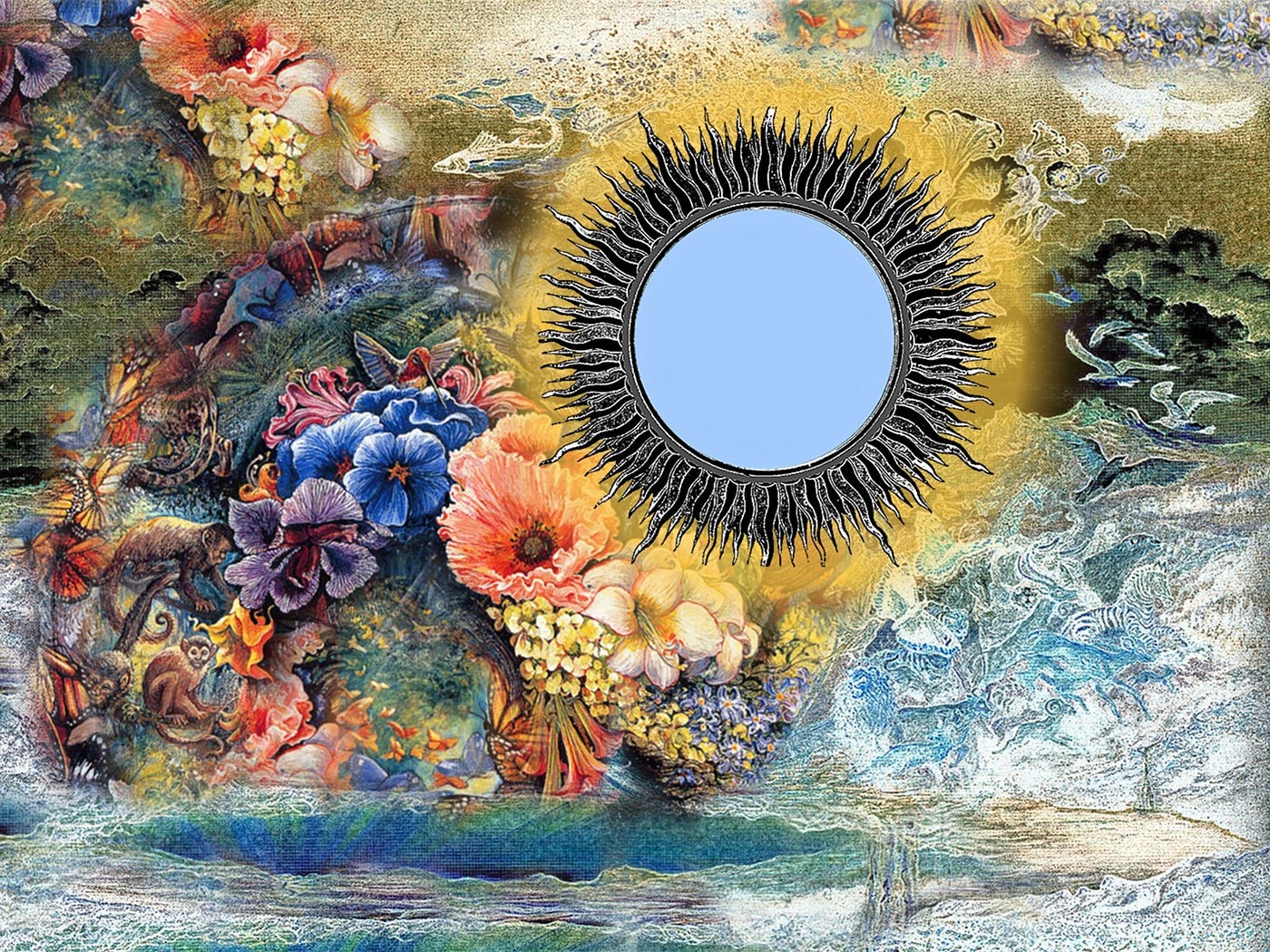This vibrant, meticulously detailed artwork, set in a landscape orientation, brims with various elements that draw the eye. Dominating the composition, just a bit up and to the right of center, is a large sun-like figure. The sun features a light blue center surrounded by black spikes, with radiant yellow shining outwards from the spikes. Below this central sun, there's a depiction of a body of water, characterized by a prominent hole and encircled by waves on the bottom right and left sides. To the left of the sun, a collage of vibrantly colored flowers and butterflies, in shades of blue, purple, pink, and yellow, mingles with clouds and images of animals. On the bottom right, the artwork transitions to a less saturated palette where a multitude of animals, appearing to be in motion, are collaged together. The careful attention to detail and rich use of color emphasize the dynamic, almost chaotic beauty of the scene, inviting viewers to lose themselves in its intricate layers.